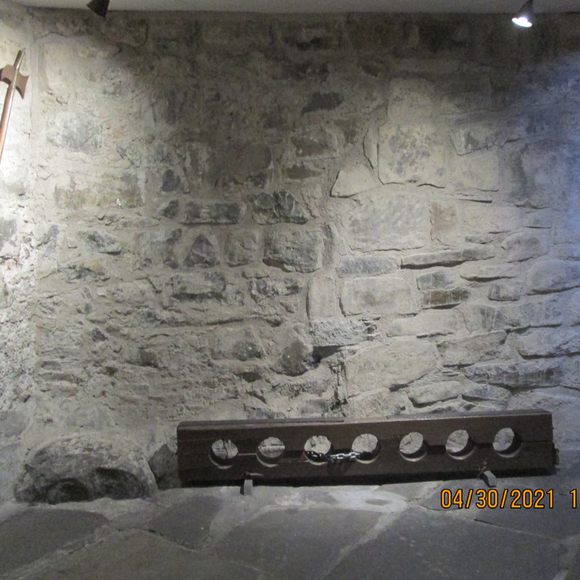This indoor photograph captures a dungeon-like scene characterized by a gray stone wall composed of varied, fitted stones cemented together and a matching gray slate floor. On the upper left corner, a metal battle axe is partially visible, mounted on the stone wall. Two white spotlights from the top illuminate parts of the wall, casting light and shadows. At the bottom of the image, a wooden block with seven holes and a metal chain threaded through two of them is placed on the floor, indicating it might be used to secure prisoners by their feet or hands. The entire setting has a monochromatic feel, with pale gray and white tones resembling a black-and-white photograph. In the photograph’s bottom right corner, the date "04-30-2021" is marked in orange digital letters, providing a timestamp for the image.